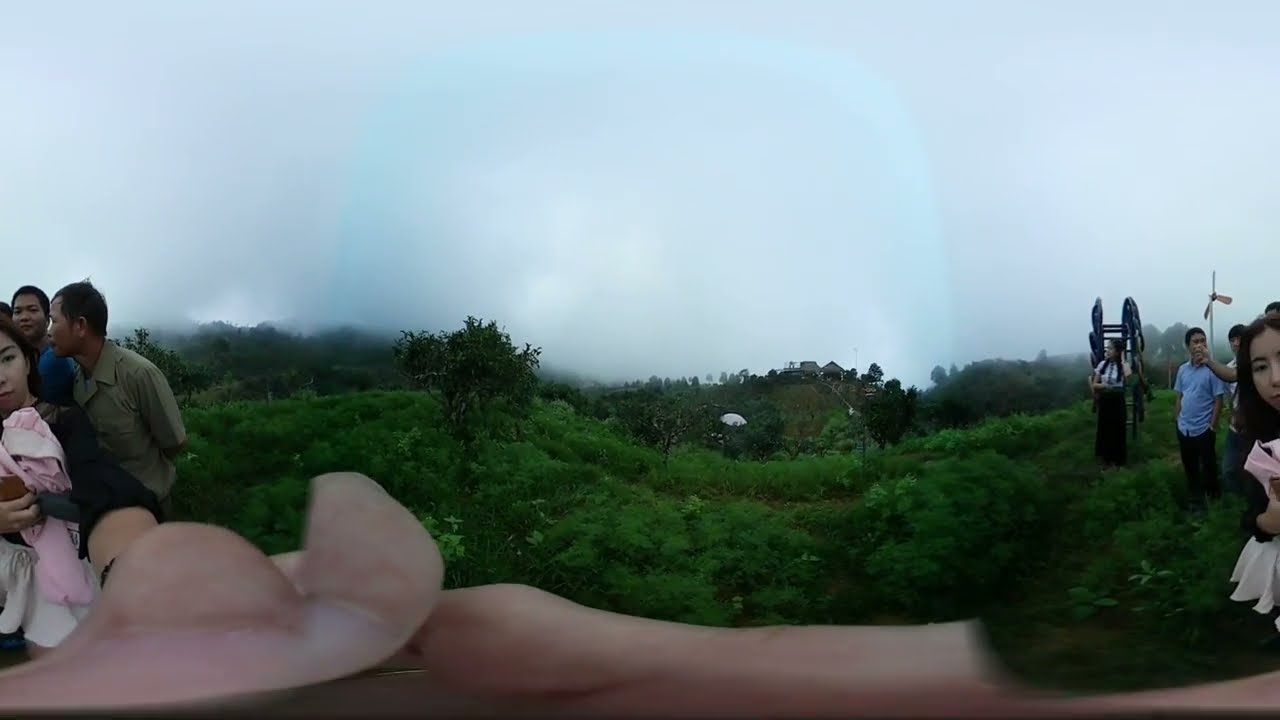This detailed photo showcases a panoramic, stitched-together image taken from a hillside overlooking a lush, green valley with a jungle backdrop. Central to the image is a woman, possibly Asian, with long brown hair, wearing a blue sleeved dress and holding an umbrella-like device in her right hand and a phone in her left. She is also seen with a pink jacket and a distinctive black ankle strip. Due to the stitching, she appears twice: split between the left and right thirds of the image.

In the left third, the woman is shown in full, accompanied by two men standing behind her and the head of a third, creating a family-like grouping. In the right third, only the right side of her face and part of her jacket are visible, alongside a man in a blue shirt with his hand raised, a visible windmill in the background, and another woman carrying what appears to be chairs or a ladder.

The central section of the panorama presents a fog-kissed hill covered in rich vegetation, with a house and a singular tree amidst the busier greeny environment. Farther down, there's a conveyance of flesh-toned distortion, possibly a thumb obscuring part of the camera lens during the stitching. Overall, this intricate panoramic image captures a mix of serene natural beauty and interesting staging quirks, possibly depicting a moment shared by a family or close-knit group enjoying the scenic overlook.